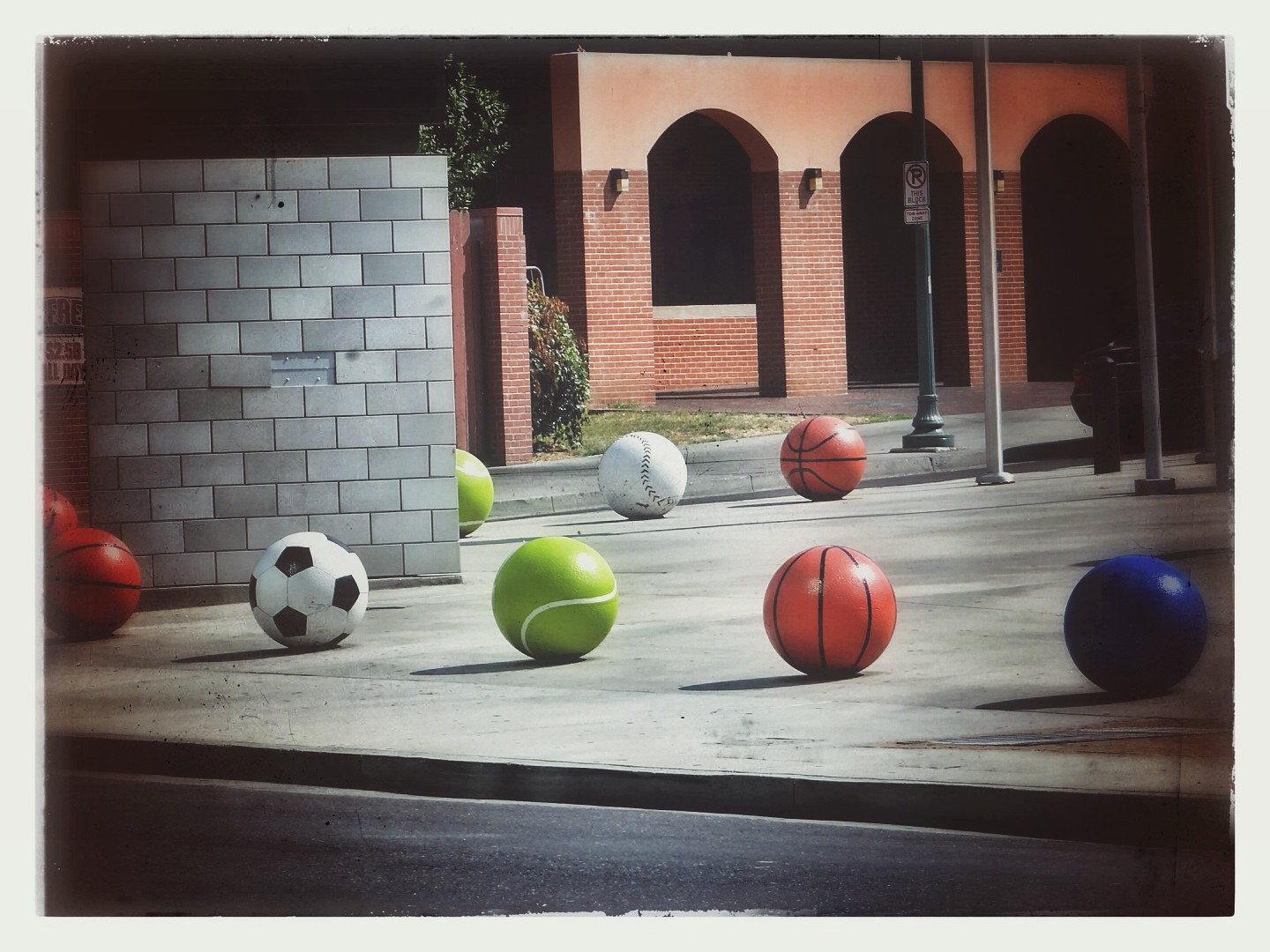An extremely wide, cement walkway dominates the foreground of the image. This pathway, approximately double the width of a standard sidewalk, is bordered at the bottom by a shaded curb and a tar roadway. Atop this unusual walkway, a series of oversized sports balls is arranged. From the middle left to the top right, there's an exaggeratedly large tennis ball, a disproportionately big white ball, and a similarly oversized basketball. Horizontally aligned at the lower section are more gigantic balls, including another basketball, a black and white soccer ball, a bright yellow tennis ball, a brown basketball, and a solid blue ball. These sports balls, each much larger than their typical sizes, appear strikingly out of place.

In addition to the sports balls, there are some infrastructural elements such as steel posts and a streetlamp with a "No Parking" sign. On the left side, a gray stone wall with darker gray grouting stands, and further back, a cinder block wall, which may be either mortared or just stacked, intersects the scene. 

Across another road in the background, a red brick building, possibly a school, features prominently. This structure has three arched doorways, each flanked by light fixtures mounted between the brick columns that transition to concrete at the tops of the arches. Visible through these arches is either a low brick wall or the side of the building, adding to the picturesque ambiance. The overall setting is adorned with curbing, grass, and well-maintained shrubs, suggesting a carefully designed, albeit surreal, environment.